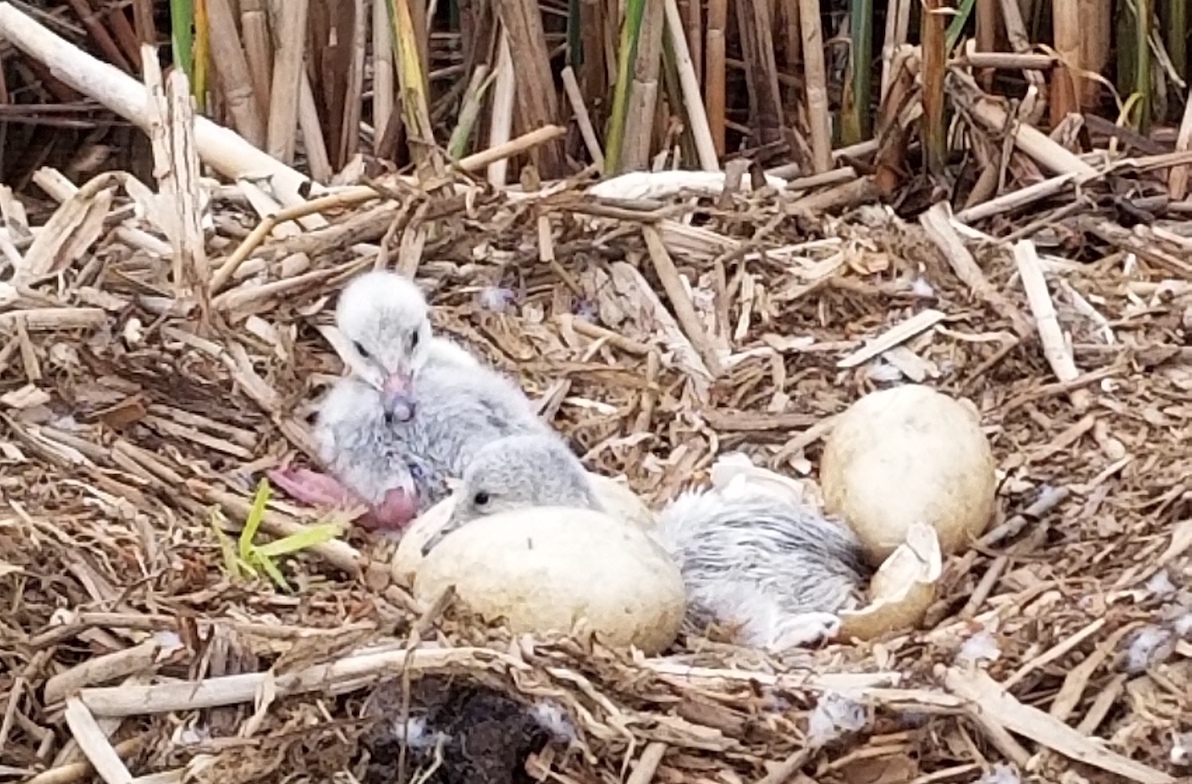This striking photograph captures a tender moment in nature, showcasing a meticulously crafted nest made of dried grass, sticks, and shredded reeds nestled among various grasses and bamboo shoots. Dominating the center of this earthy bed are two fluffy, newly hatched baby ducklings with soft grayish-white feathers, one of which is slightly scruffy in appearance. The ducklings, with their pink feet tucked beneath them, are accompanied by a mix of hatching activity, including two to three unhatched creamy white eggs and fragments of thick eggshells nearby, suggesting imminent action. In the background, a blend of brown, dying reeds interspersed with a few green ones adds a rich texture to the scene, emphasizing the natural habitat. Captured without any parent ducks in sight, this image powerfully depicts the fragile yet awe-inspiring beginning of new life.